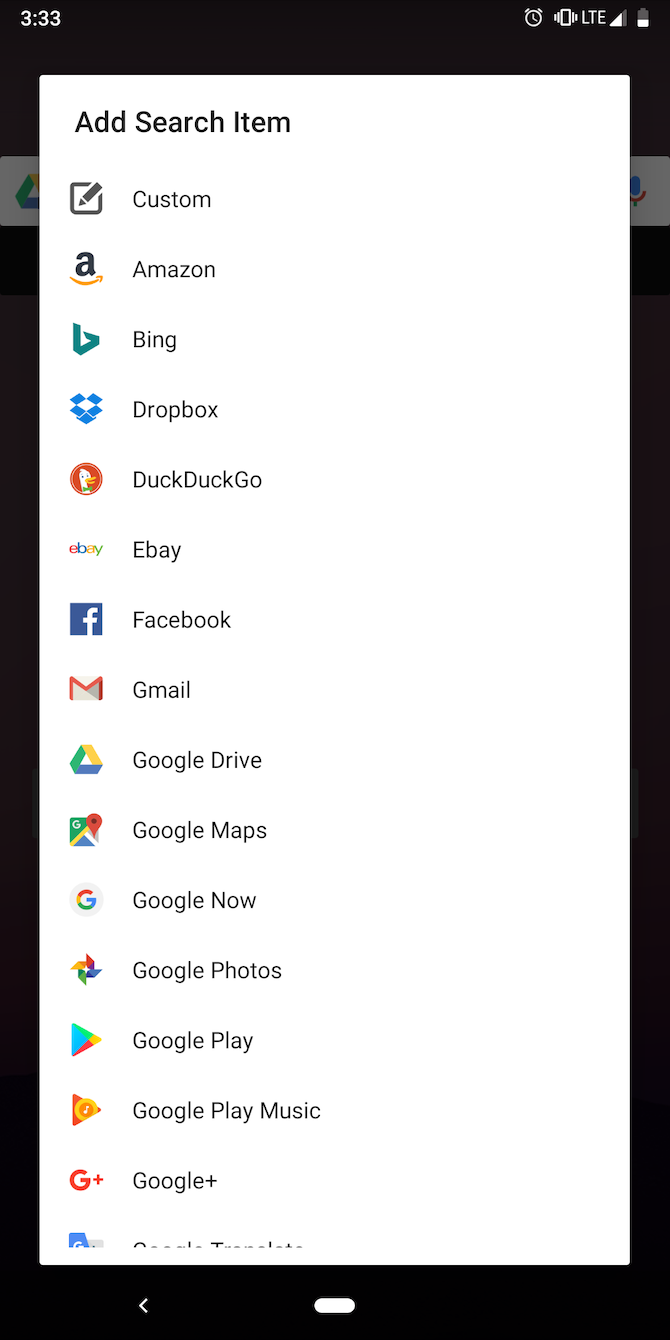This is a detailed caption for an image showing a screenshot taken on a smartphone:

"Screenshot of a smartphone displaying an interface with various app options. The top left corner shows the time as 3:33, and the top right corner displays a battery icon that is slightly less than half full. Below these indicators, there is a pop-up window titled 'Add Search Item' in black text. Under this heading, a list of apps is shown in alphabetical order: Custom, Amazon, Bing, Dropbox, DuckDuckGo, Ebay, Facebook, Gmail, Google Drive, Google Maps, Google Now, Google Photos, Google Play, Google Play Music, and Google Plus. The bottom of the list is slightly cut off, but 'Google Translate' is partially visible. The apps listed appear to include search engines, social media platforms, email, cloud storage, and various Google services, suggesting that the user has a diverse range of apps installed and uses multiple browsers — Google, DuckDuckGo, and Bing."